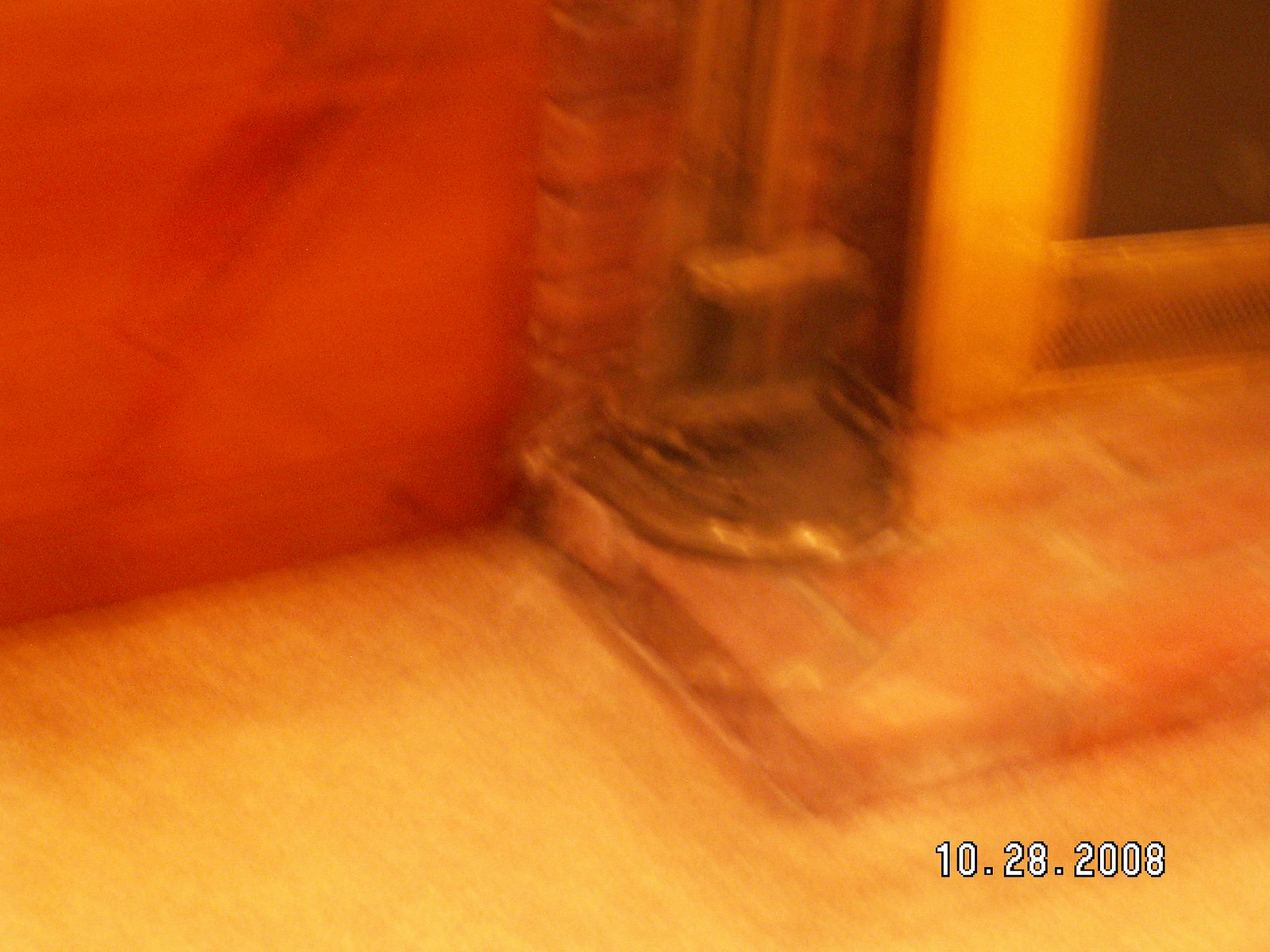This blurry photograph, taken on October 28, 2008, depicts part of a building's exterior or possibly an interior space with a doorway. The image features a red brick wall, with visible grout lines, that forms a corner with a ledge made of similar red brick. The flooring appears to have an off-white or light yellow hue. There is a mysterious metallic object, resembling a horseshoe or arch shape, which could potentially be part of a door frame, a drain lid, or the surrounding of a fireplace. Additionally, a gold-colored metal object, possibly a door with hinges, is situated near the brick structure. The photograph has a stamp at the bottom right corner, reading "10.28.2008." Despite its blurriness and graininess, detailed features such as the brick pattern and grout can still be discerned.